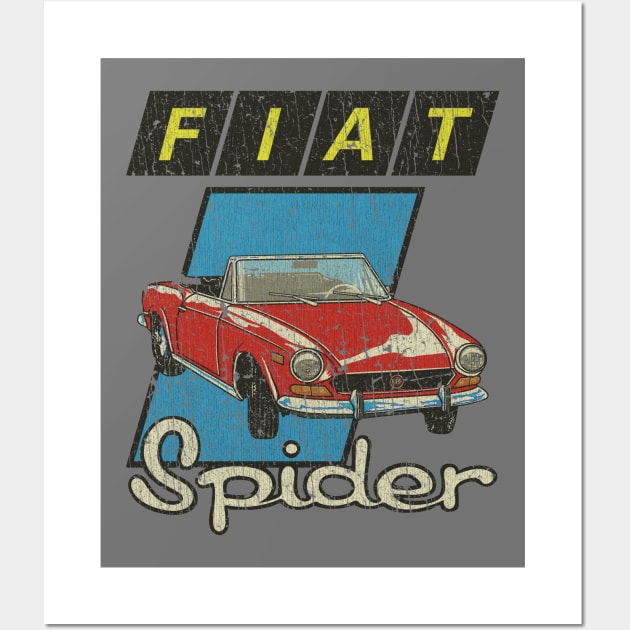The image is an advertisement for the Fiat Spider, set against a light gray background with a sleek design. At the top, the word "FIAT" is prominently displayed in yellow italic letters, each enclosed in its own slanted black box. Below the lettering, the central focus is a detailed illustration of a vintage red Fiat Spider convertible, with the top down and black tires. This classic car features white trim around the bumper and windows, adding to its distinctive look. Behind the car, a stylish blue trapezoid with a black outline enhances the visual appeal. At the bottom of the image, the word "SPIDER" is elegantly written in a cursive script, adding a touch of sophistication to the overall design. This visually striking poster exudes a sense of nostalgia and elegance, making it a perfect piece for any car enthusiast's collection.